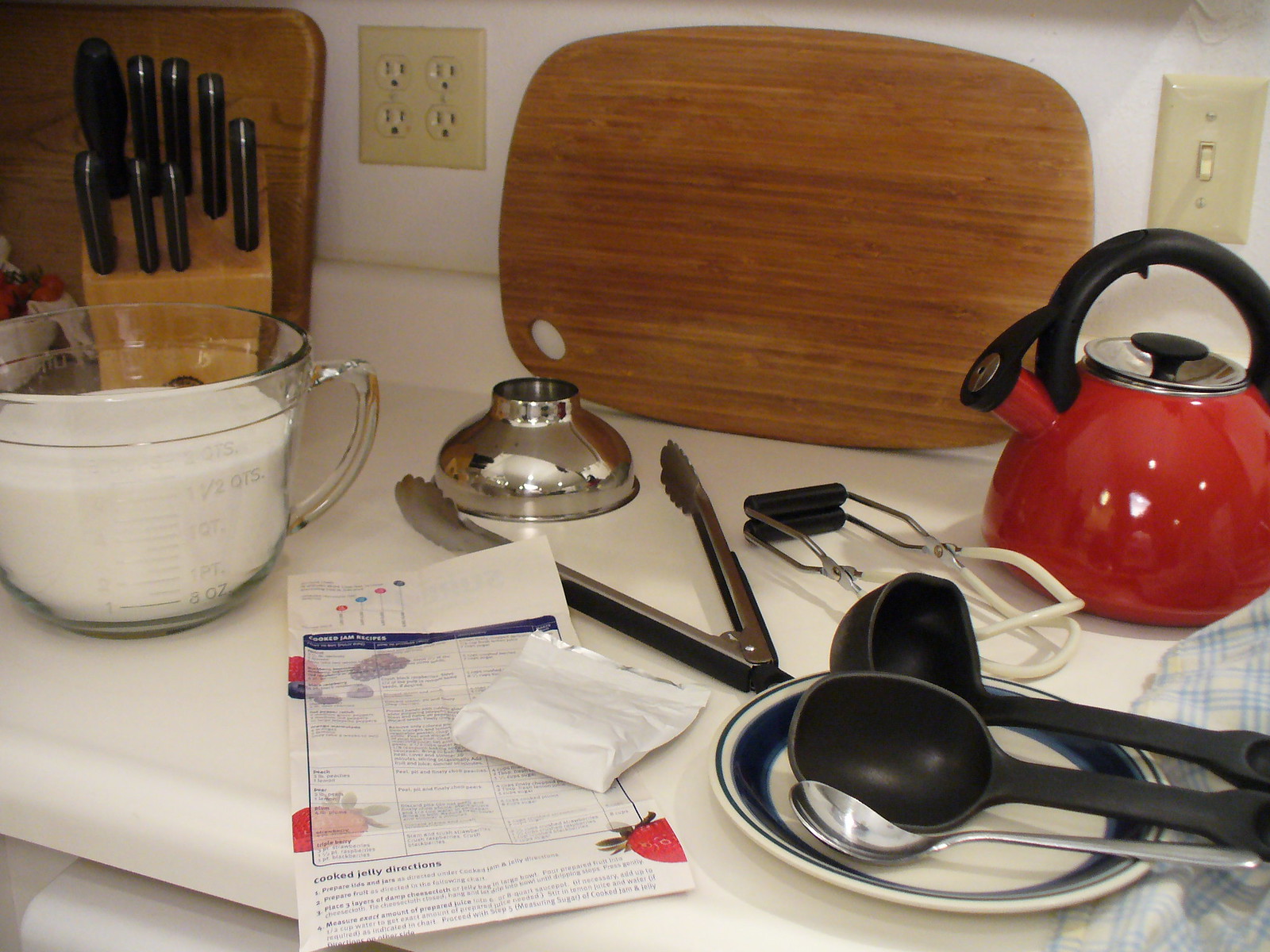Close-up view of a kitchen countertop showcasing an ongoing canning process. The countertop is a white or off-white Formica with a four-inch backsplash. Several cutting boards are propped up against the wall. A beige four-hole wall outlet and matching light switch are visible nearby. The countertop displays a red tea kettle, a large glass measuring cup filled with ingredients, likely next to a bowl of strawberries in the background. 

A wooden knife block holds seven knives and a sharpening rod. A recipe featuring strawberries suggests the canning theme. Essential canning tools, including a stainless steel funnel, stainless steel and black tongs, and a jar lifter, are laid out. Cooking utensils like a stainless steel spoon, two black nylon spoons, and a ladle rest on a white saucer with black rings. A blue and white check tea towel is placed under the handles of the spoons.